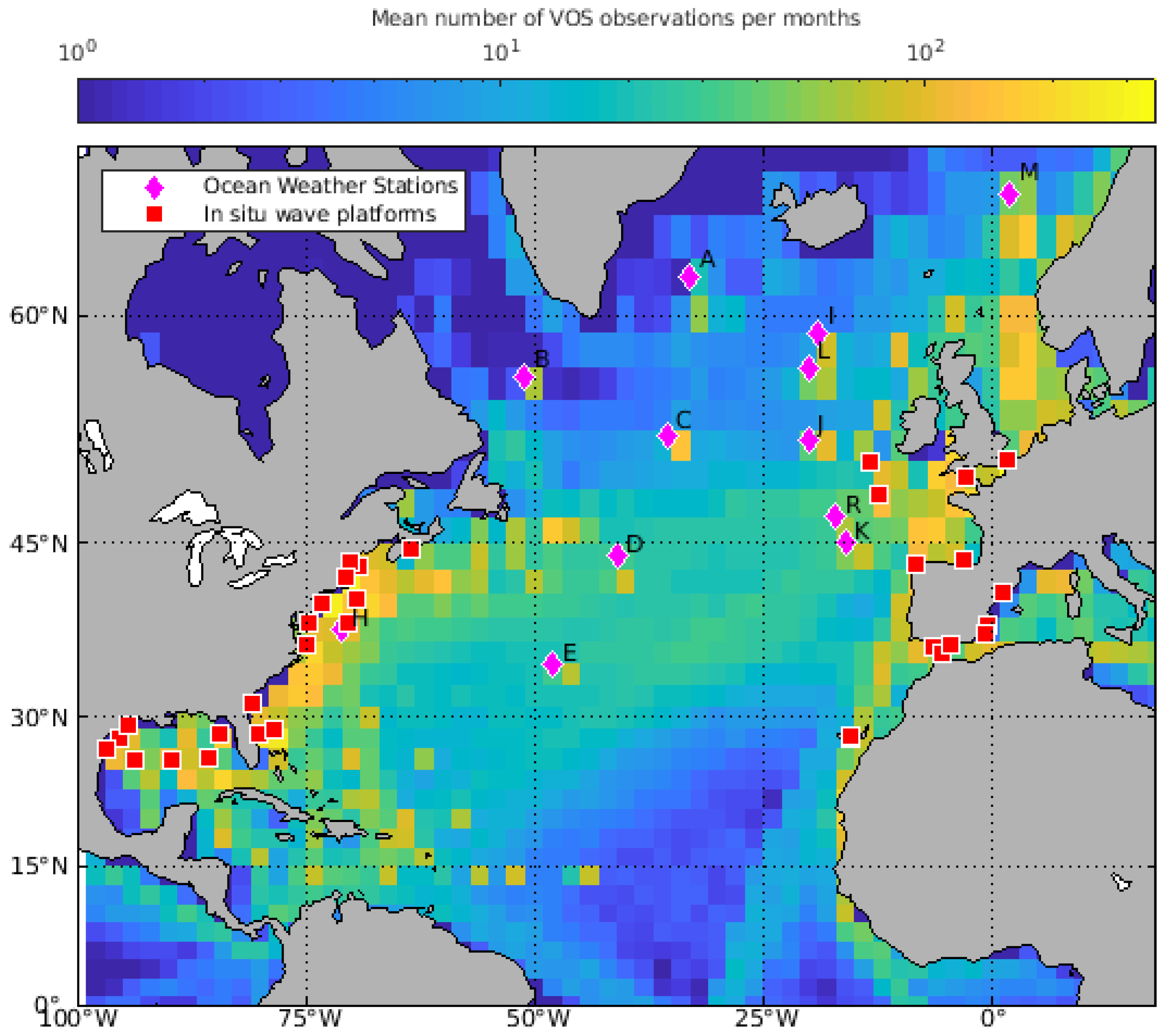This image depicts a detailed weather pattern map reminiscent of those seen on the Weather Channel or similar to Doppler radar images. The map is vertically oriented with a white background. Across the top, there's a horizontal bar labeled "mean number of VOS observations per month," starting from "10-0" on the left, progressing through "10-1" in the center, and ending at "10-2" on the right. This bar transitions in color from dark purple to dark blue, light blue, and finally to an orangey-yellow and yellow as it moves from left to right.

Below this, a large, gray-rectangled area forms the background for a prominent landmass centrally located, which notably resembles the shape of a frog with its legs splayed out. This landmass is composed of various colors, including dark blue, light blue, greens, yellows, and oranges, arranged in a grid-like pattern. Scattered across the map are numerous red squares and purple diamonds, identified in a key at the top as in-situ wave platforms and ocean weather stations respectively.

The map includes detailed grid lines for longitude and latitude, marked on the left from 0 to 60 degrees North and at the bottom from 100 degrees West to 0 degrees West. Dotted lines extend horizontally and vertically from these grid markers. Additionally, the map features the recognizable outlines of the state of Michigan and the surrounding Great Lakes on the lower middle left, enhancing its geographical context.